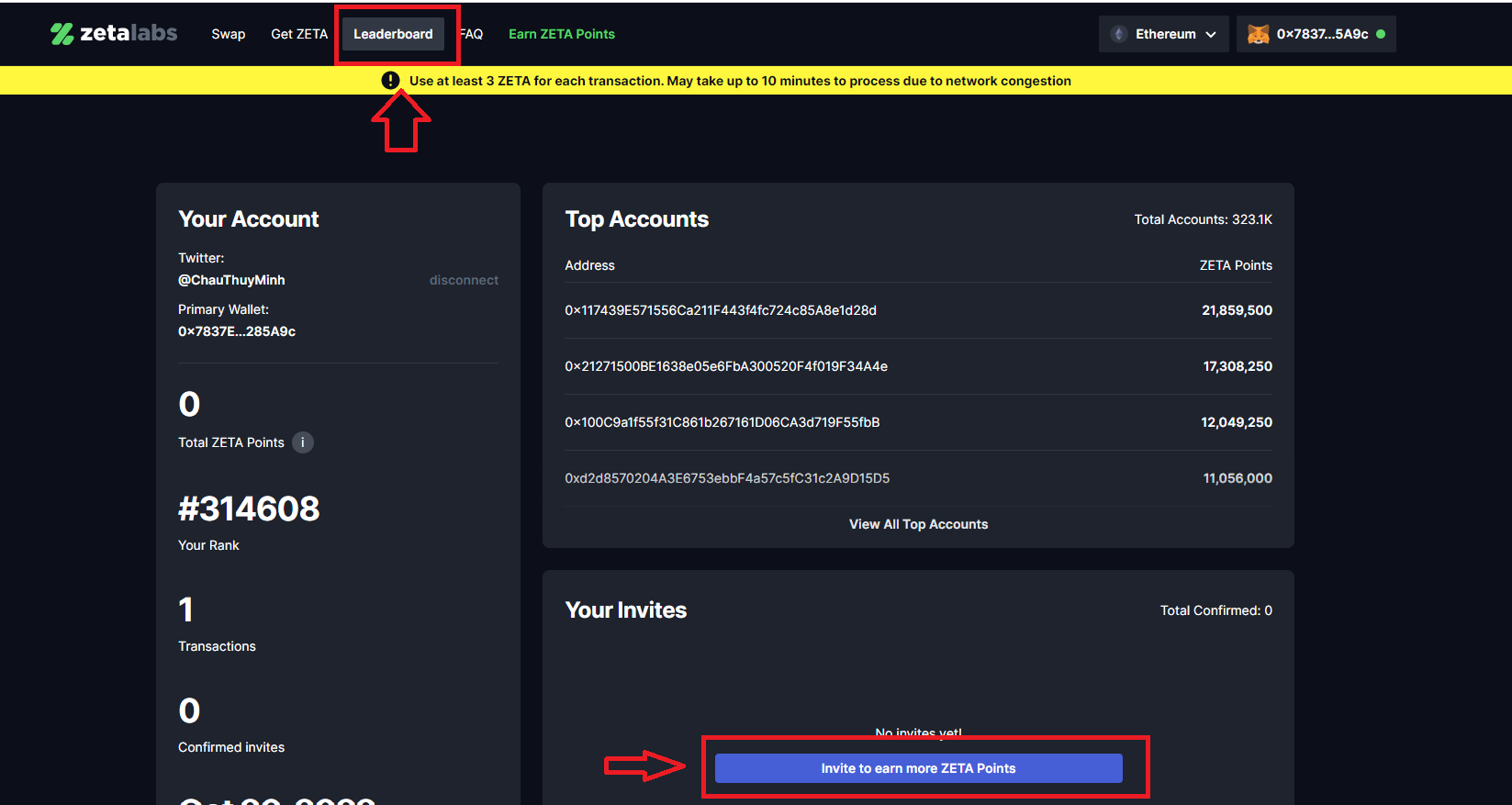The screenshot showcases the web page of Zeta Labs with a distinctive layout and several interactive elements. 

In the top left corner, the logo is prominently displayed featuring a green percent icon, followed by the text "Zeta Labs." The word "Zeta" is in white, while "Labs" appears in gray. The navigation menu includes buttons labeled "Swap," "Get Zeta" (in all capitals), "Leaderboard" (highlighted in a red box), "FAQ," and "Earn Zeta Points."

On the far right of the header, there is a tab labeled "Ethereum." Adjacent to this, a digital code is displayed, preceded by a wolf icon. The code reads "0x78375A9C," and next to it, a green dot indicates the online status. 

Beneath the header, a yellow rectangular bar advises users: "Use at least three Zeta for each transaction, may take up to 10 minutes to process due to network congestion."

The main content of the page is divided into sections. The first section labeled "Your Account" contains various details about the user's account. Adjacent to this, another column titled "Top Accounts" lists addresses of the leading accounts. Further down, there is a section for "Your Invites," indicating the user's referrals.